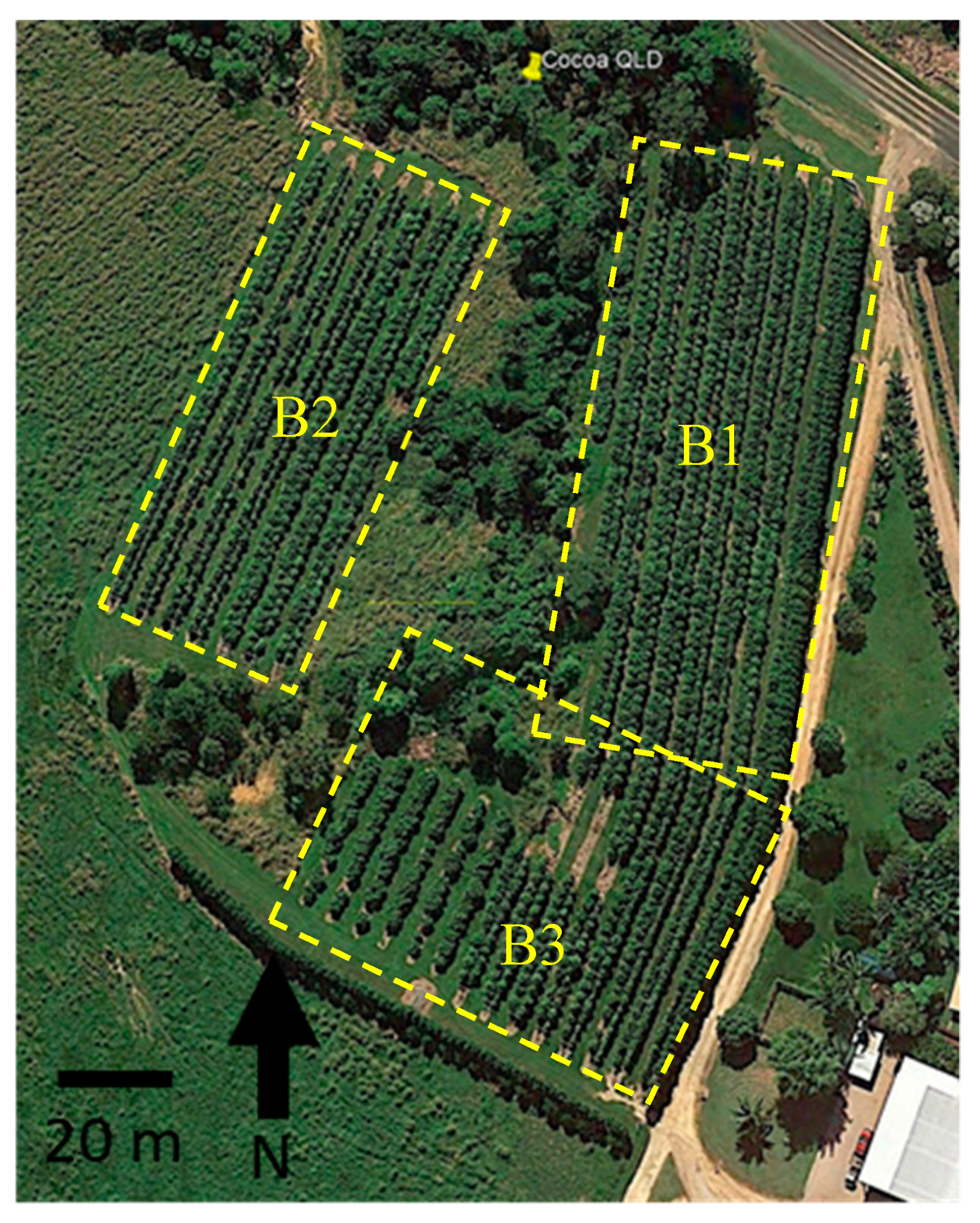This detailed aerial view photograph captures a serene countryside landscape with three distinct rectangular plots of agricultural land, prominently outlined with broken yellow lines. The plot labeled B2, located in the upper left, has approximately eight or nine rows of planted crops and is shaped like a rectangle extending from the bottom up to the right. Adjacent to B2, to the right, is plot B1, which is a more upright rectangle featuring nine or ten rows of similar-looking crops. Below B1, there is the shorter, broader plot B3, containing six short rows of crops on the left and ten longer rows on the right. 

A mixture of open ground, dirt, and patches of grass lies to the left of B2, while clusters of trees fill the spaces above the plots and between B2 and B1. A dirt road in the upper right corner extends diagonally across the image; it curves from the upper right to the middle right and continues downward, finally bending at the bottom towards a small white building in the bottom right-hand corner. 

B3 borders more clusters of trees and bushes toward its left. Additionally, the bottom left-hand corner of the image features a scale indicator of 20 meters and a direction arrow pointing north. The aerial view provides an insightful representation of orderly structured agricultural fields interspersed with natural elements, all connected by a network of dirt paths.